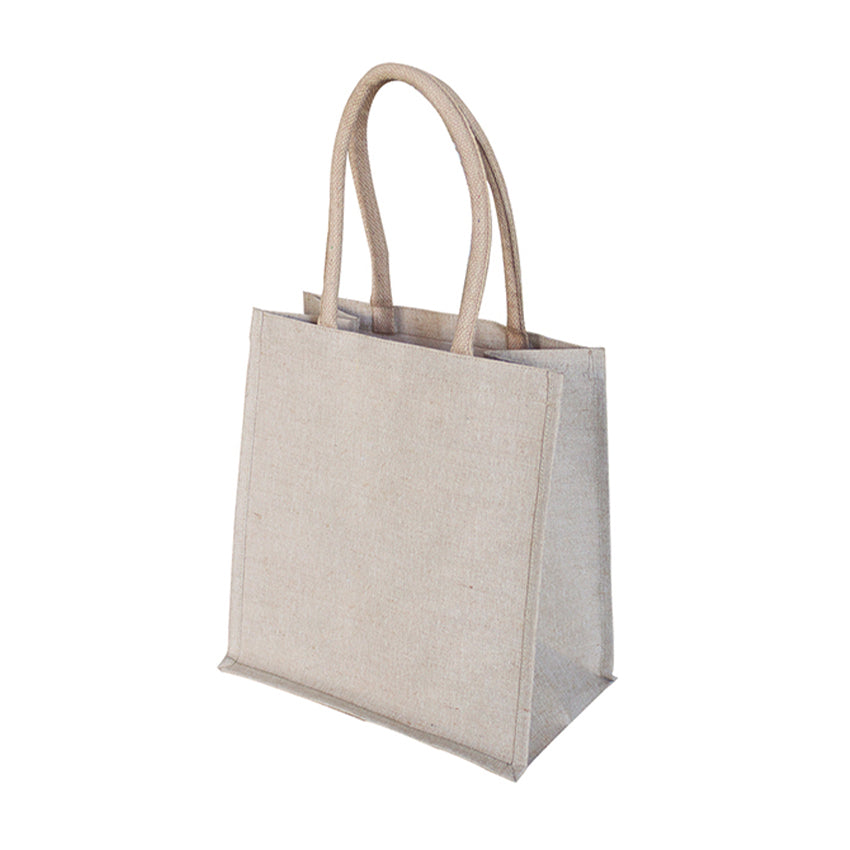The image showcases a light gray, almost beige, canvas tote bag against a stark white background. The bag is square-shaped, with noticeable details such as its flat base, which suggests it has some internal support, possibly cardboard, to prevent it from toppling over when set down. The handles are a prominent feature, appearing to be rolled and padded, potentially made from faux leather or rope-like material, providing a comfortable grip. The bag is slightly open, with its sides folded inwards, hinting that it is empty. It has square corners and visible lining, contributing to its structured appearance. The overall style is basic and functional, designed to resemble reusable grocery bags, ideal for everyday use. There is no text present within the image.